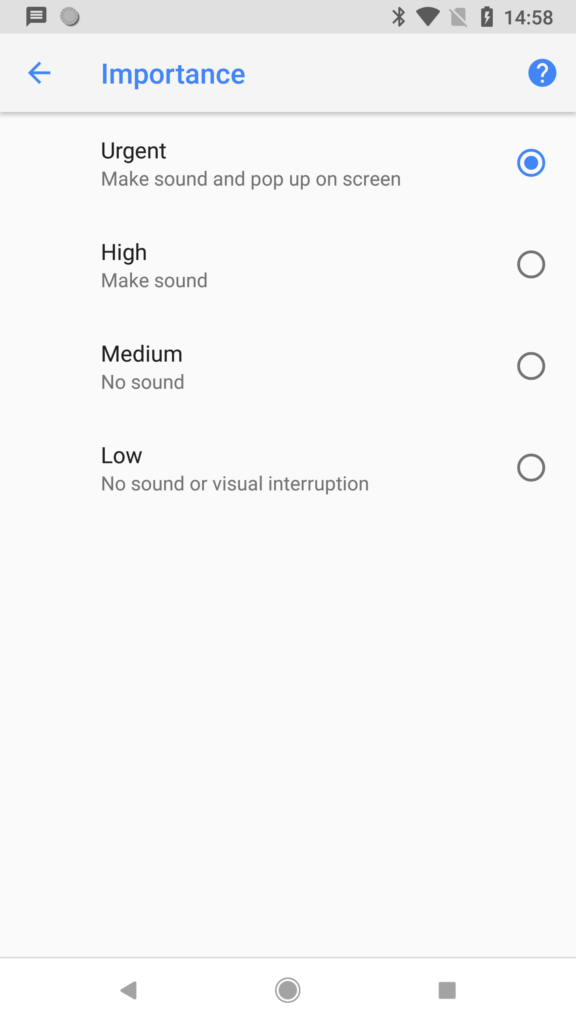A smartphone screen showing an app's notification settings interface. The app appears to allow users to customize the importance of notifications. The "Importance" setting, prominently displayed in blue, differentiates four levels of notification priorities: "Urgent," "High," "Medium," and "Low." Each level is accompanied by a brief description. Currently, "Urgent" is selected, indicating that notifications will generate a sound and a pop-up on the screen. The other settings include "High" for sound-only notifications, "Medium" for silent notifications, and "Low" for notifications without sound or visual interruptions. A back button is visible at the top-left corner, while a question mark icon near the "Importance" title likely links to additional information. The background of the app is gray, and most text is rendered in black. Additionally, the phone’s status bar shows an unread message, a full battery that's still charging, full Wi-Fi, and a Bluetooth connection.